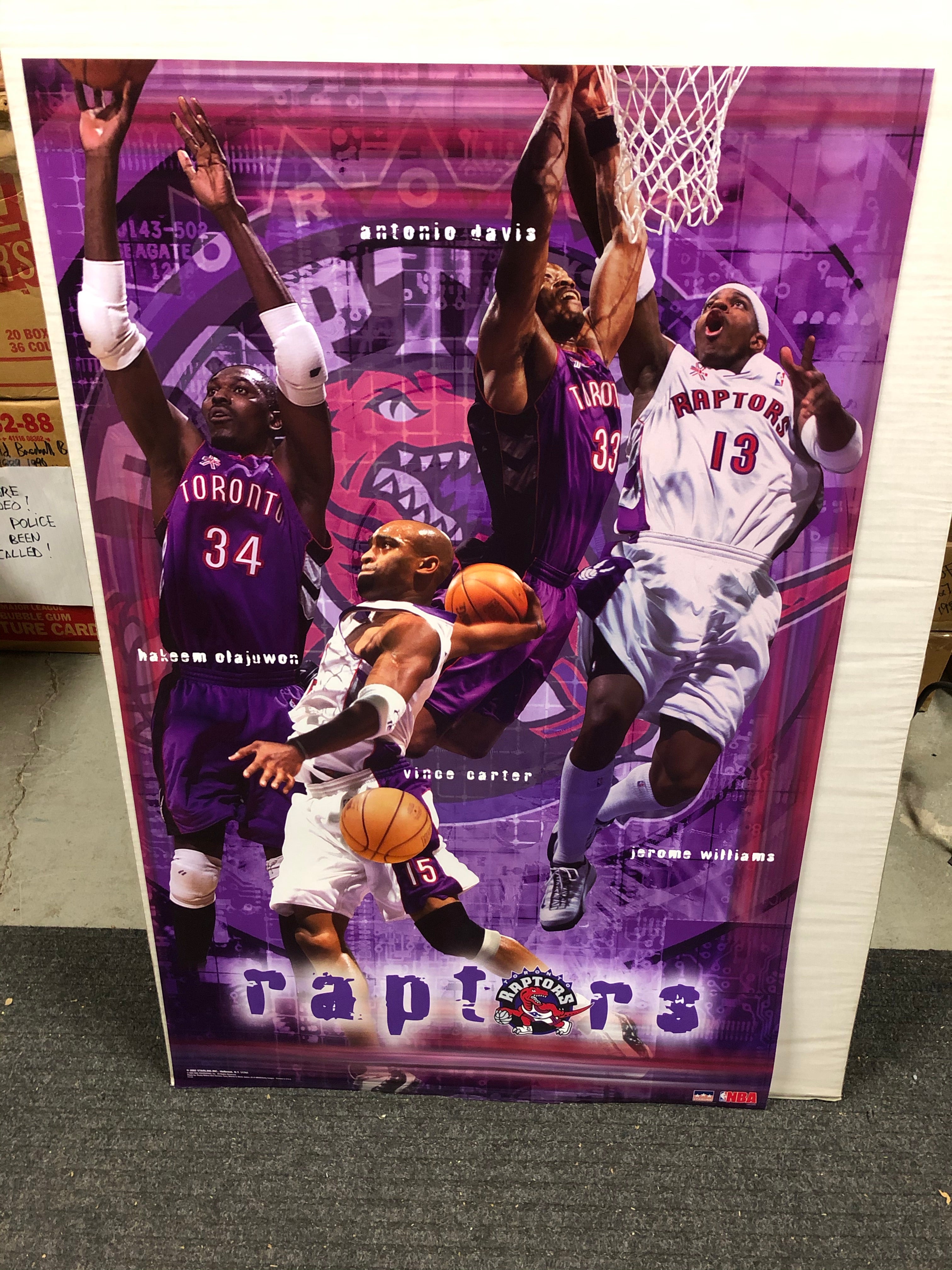The image is a photograph of a poster advertising the Toronto Raptors basketball team. The poster, which appears to be around five to six feet tall, is lying on a gray rug or carpet and is bordered by a white cardboard frame. Behind the poster are several cardboard boxes with red print, and the floor features a visible crack. The poster itself has a vibrant purple background and prominently displays the Raptors' logo, a cartoon drawing of a raptor. Four African-American basketball players are captured mid-jump: two in purple jerseys and shorts with the numbers 33 and 34, presumably Vince Carter and Antonio Davis; and two in white jerseys and shorts with the numbers 13 and 15, with Hakeem Olajuwon being the noticeable name. The players are depicted in various dynamic poses, with one of them shooting into a basketball hoop. The players' names are written in white text. Other colors that stand out in the poster include red, pink, orange, and brown, contributing to the vivid and eye-catching design.